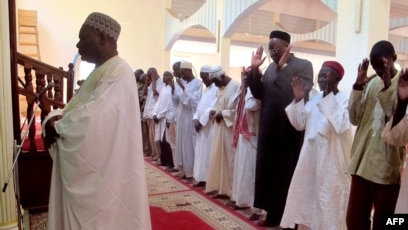The image depicts a religious ceremony inside a grand place of worship, characterized by its tall white columns, intricate woodwork, and ample windows. In the foreground to the left stands an African American man, presumably leading the ceremony, adorned in a long white robe that reaches the floor, and a snug, crocheted or yarn-made hat resembling a turban. This figure is slightly turned towards a wall area with a post. To his right, a line of African American individuals, some in similar white robes and others in suits, stand solemnly on a red rug. Their hands are raised, possibly in prayer, and their eyes are closed, signifying a moment of deep reverence. These individuals also wear fitted white hats. In the background, under large arches, a wooden railing is visible, indicating stairs within this spacious and sacred setting, suggesting a sense of unity and collective worship among the participants.